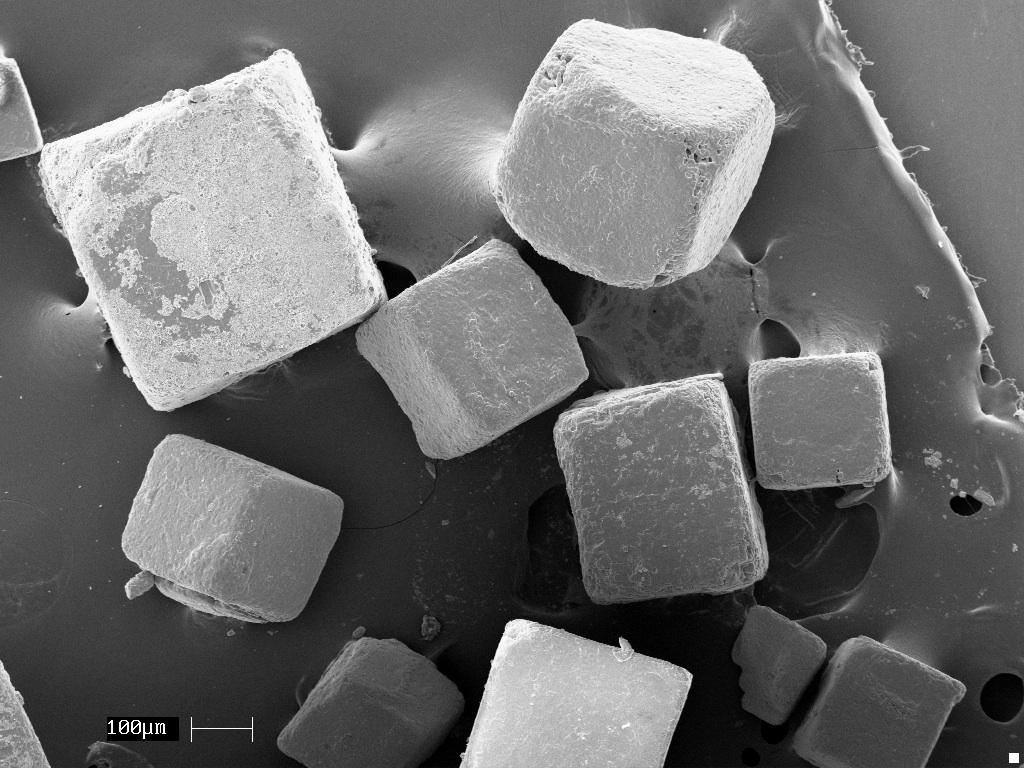This black and white photograph features an array of scattered cubes of varying sizes and textures on a flat, stony gray background. The image is marked with the text "100 UM" in white at the bottom left corner. These cubes appear to be made of stone or cement, although some interpretations suggest they could resemble marshmallows or powdered jelly candies due to their irregular shapes and broken corners. The cubes are predominantly gray and white, but there are darker gray ones at the bottom. The arrangement of the cubes is seemingly random, with a prominent white cube in the upper left and a uniquely shaped, almost marshmallow-like cube beside it.